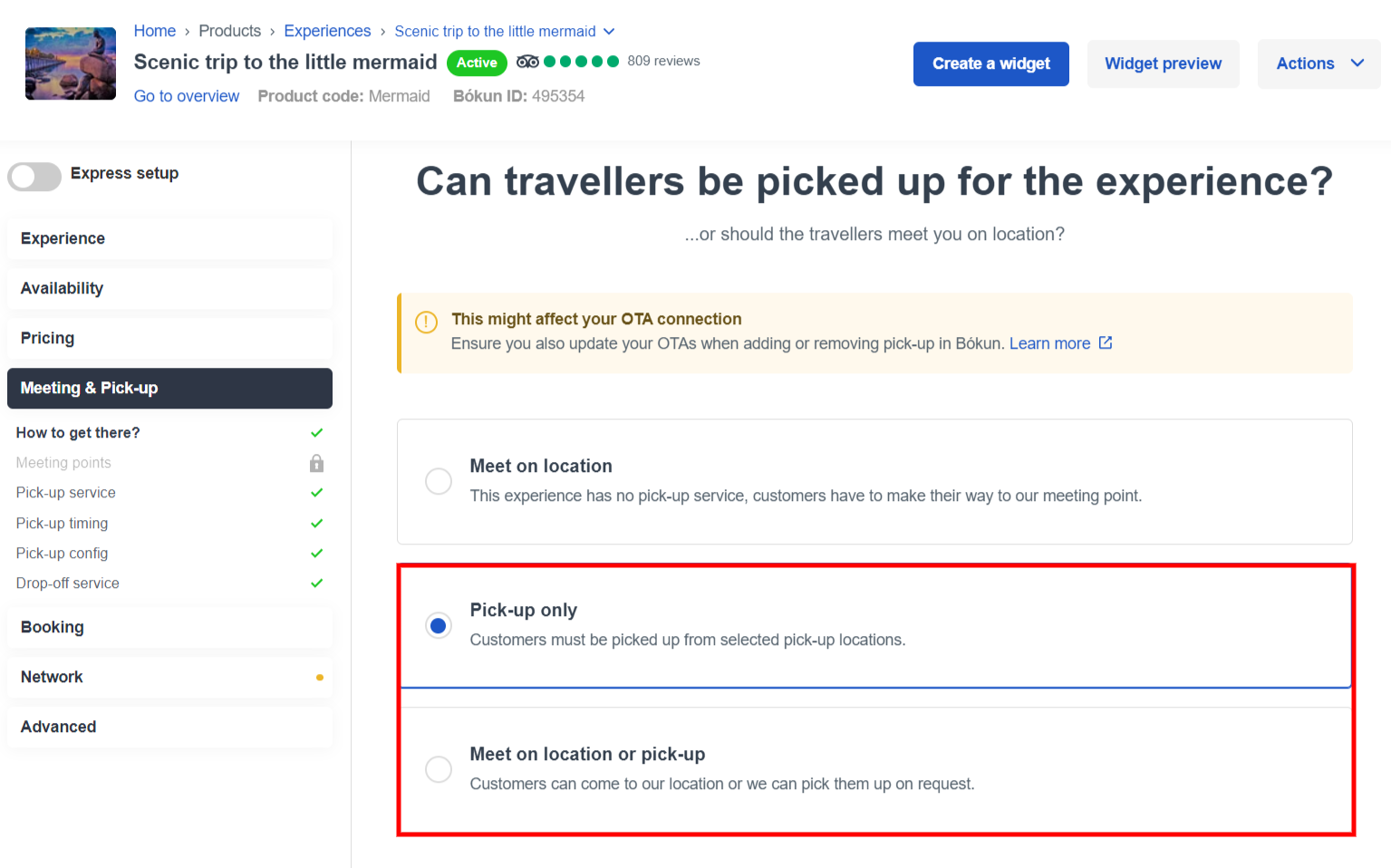In this image set against a white background, there is a header with a few prominent features. On the left side of the header is an illustration of a mermaid sitting on a rock by the water. To the right of the illustration, in dark gray text, are the words "Scenic trip to the Little Mermaid." Further to the right, there is a button labeled "Active" in white text. Below the button is a five-circle TripAdvisor rating with "809 reviews" indicated. Underneath, in blue text, it says "Go to overview," and next to it in gray text, it reads "Product code: mermaid."

Below this section, bold text poses the question: "Can travelers be picked up for the experience?" In smaller lowercase text beneath it, it asks, "or should the travelers meet you on location?" 

Outlined in a red border are two options for the pickup arrangement. The first option, labeled "Pickup only," states that "Customers must be picked up from selected pickup locations" and is marked with a blue circle indicating its selection.